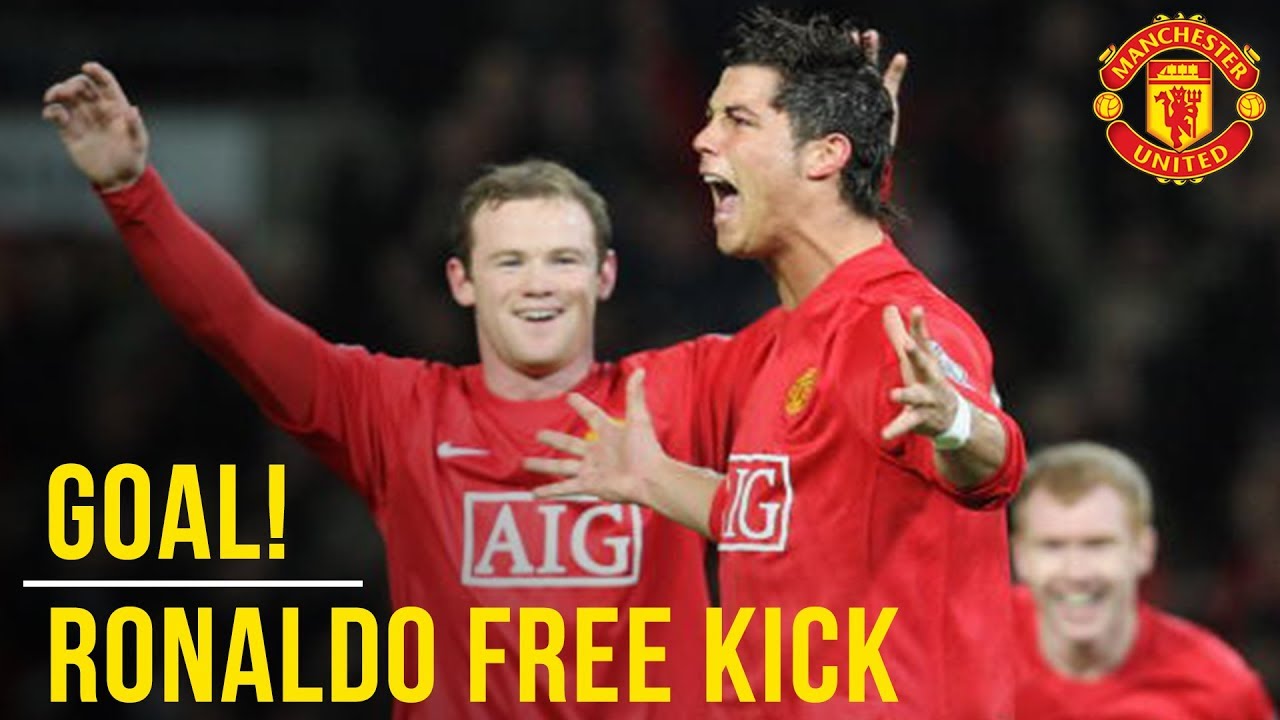The photograph captures a thrilling moment of celebration featuring three male soccer players wearing red long-sleeved Manchester United jerseys with white "AIG" lettering in the center. The main focus is on two players: the one closest to the camera is turned to the side with his arms outstretched, and the player behind him is fully facing the camera with his arms raised and a look of intense excitement, his veins visibly protruding from his neck as he appears to be shouting. In the background, a third, slightly blurred player is seen crouched down, also celebrating joyfully. The background is dark and out of focus, possibly indicating a night game or an indoor setting. In the bottom left corner, the text "GOAL! Ronaldo Free Kick!" is prominently displayed in yellow, separated by a white line. The top right corner features the "Manchester United" name and logo in red and yellow, adding a sense of team pride to the image.